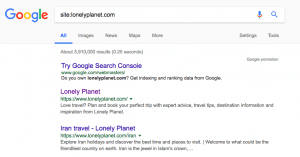This image is a screenshot from the Google search engine results page. At the top left, the familiar Google logo is prominently displayed, featuring the blue "G," red "O," yellow "O," blue "G," red "E," and green "L." The search term used is "site:lonelyplanet.com." 

The results begin with an advertisement that encourages users to "Try Google Search Console." Directly beneath the ad, the primary result for the website Lonely Planet appears. The listing reads "lonelyplanet.com," followed by a brief description of the site. The specific result highlighted is titled "Iran Travel – Lonely Planet." The accompanying description states, "Explore Iran holidays and discover the best time and places to visit."